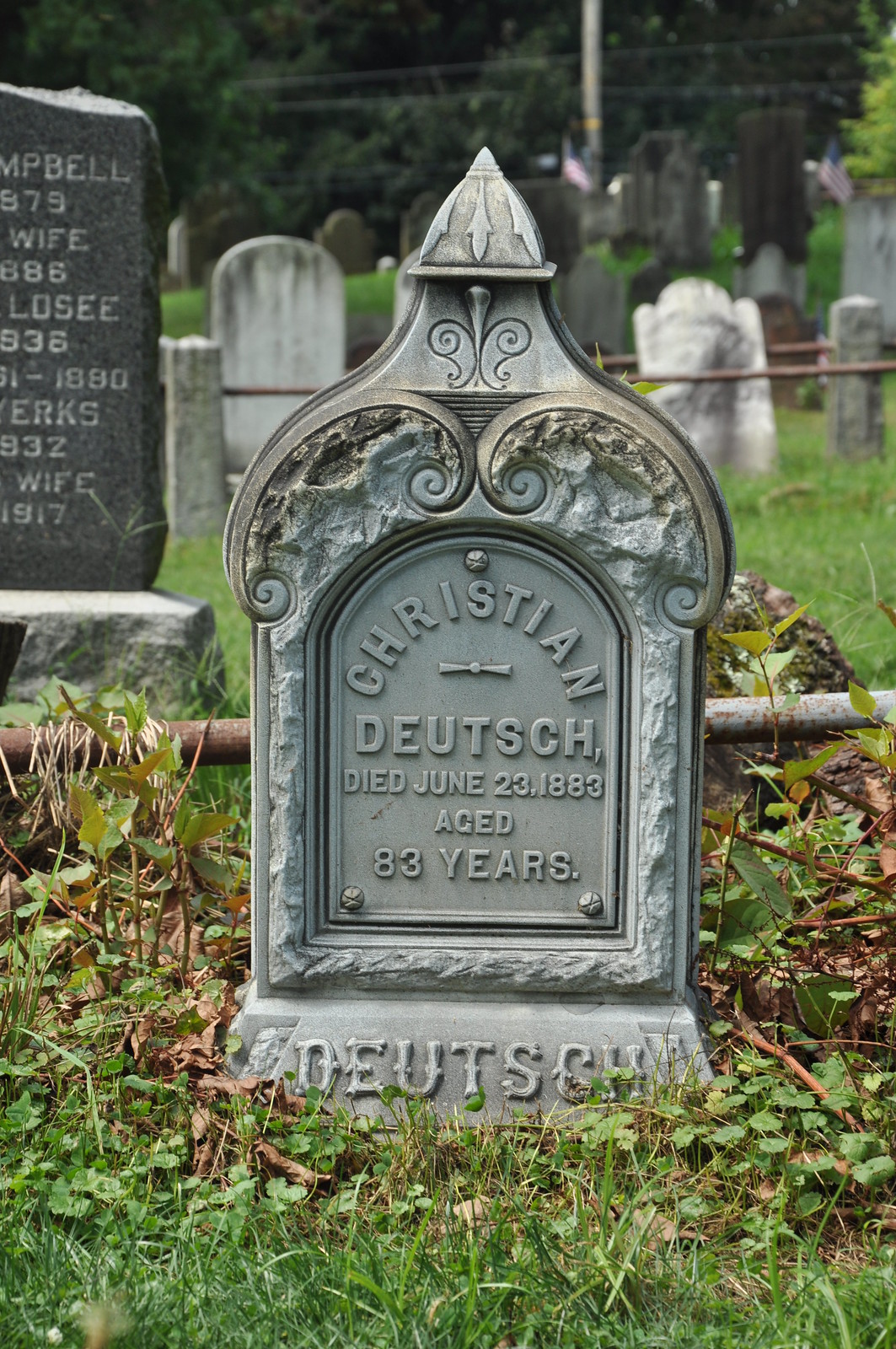The image captures a serene daytime scene of an old cemetery, with the focal point being a beautifully intricate, light gray tombstone of Christian Deutsch. The headstone is prominently inscribed with "Christian Deutsch" in a half-circle shape at the center, and below that, it reads "Died June 23rd, 1883, aged 83 years." The tombstone's structure is distinctive, featuring a flat bottom that curves inward towards a pointed top, adorned with intricate designs along the edges. The gravestone is positioned in a lush grassy area with green leaves flourishing around its base, indicating it has been there for a considerable time. Directly behind the headstone lies a rusted bar on the ground, with more weathered and diverse headstones further back. These vary in material and color, ranging from simple rounded stone markers to black marble gravestones, some with visible inscriptions while others are obscured by time. The backdrop is dominated by a dense row of dark green trees, among which a single silver pole and a few power lines are visible, subtly hinting at a nearby road. The peaceful seclusion of this cemetery is further emphasized by the presence of American flags and minimal signs of modern encroachment, lending a timeless quality to the scene.